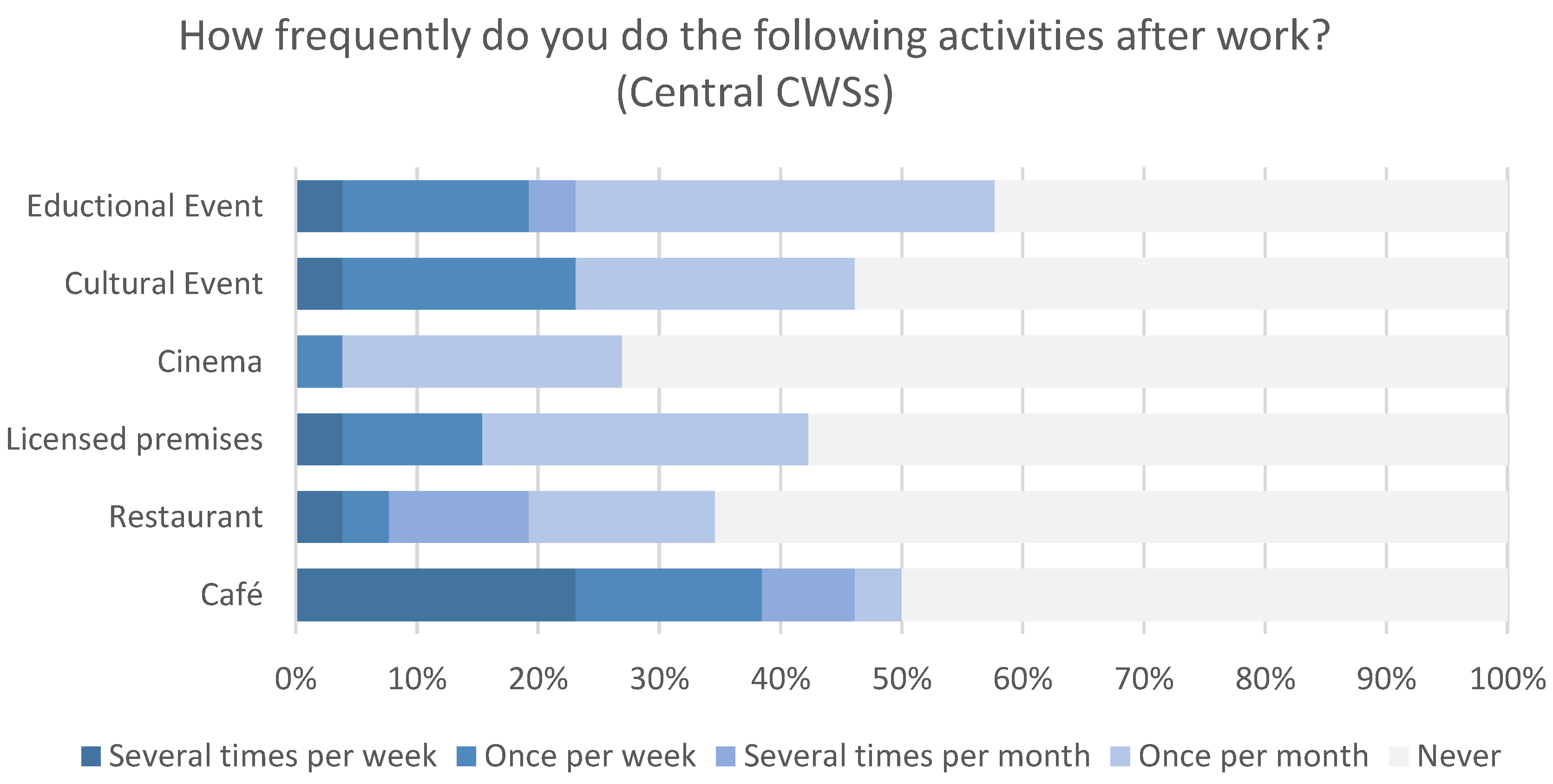This image features a detailed line graph titled "How Frequently Do You Do the Following Activities After Work?" with the note "central CWSS" in parentheses. The graph analyzes the frequency of participation in various after-work activities such as educational events, cultural events, cinema, licensed premises, restaurants, and cafes. 

The x-axis of the graph ranges from 0% to 100% in 10% increments, while the y-axis categorizes the activities. A color-coded key at the bottom of the graph indicates the frequency of these activities: several times per week, once per week, several times per month, once per month, and never.

According to the graph, the participation rates are as follows: educational events peak at approximately 58%, cultural events at around 48%, cinema at 28%, licensed premises at 42%, restaurants at 33%, and cafes at 50%. Each category is represented with varying shades of blue to depict the different frequencies of engagement.